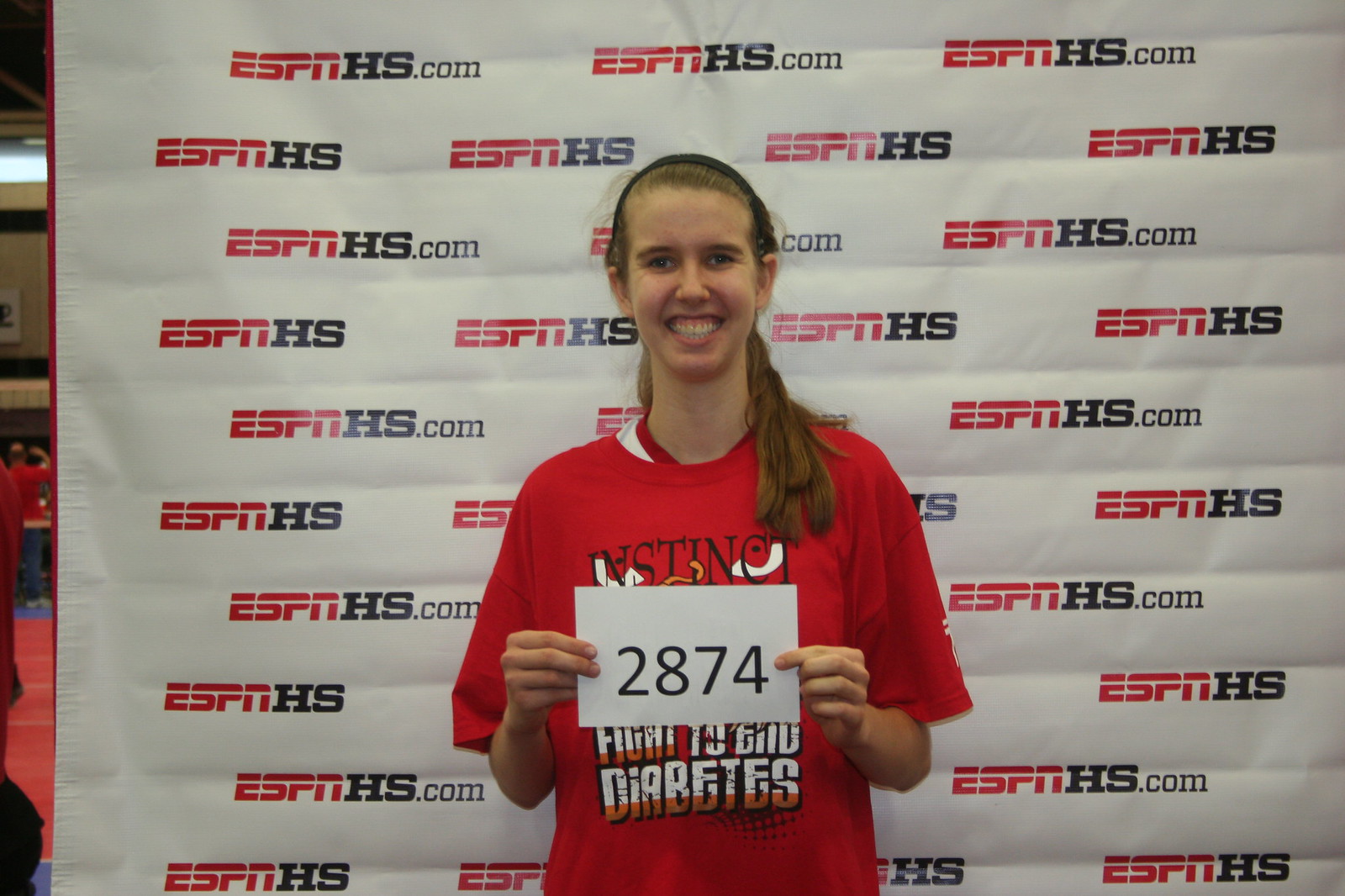This indoor photograph, measuring approximately 6 inches wide and 4 inches tall, features a high school girl of Caucasian descent standing in front of a prominently displayed ESPNHS.com banner. The white banner is adorned with "ESPN" in bold red lettering and "HS.com" in black, repeated both horizontally and vertically across the background. The teenage girl, likely around 15 or 16 years old, has long brown hair styled in a ponytail over her left shoulder and a black headband securing her hair away from her forehead. She is wearing an oversized red T-shirt that reads "Instinct, Fight to End Diabetes" and appears to have another red T-shirt underneath. With a broad smile directed at the camera, she holds up a white placard bearing the number 2874 with both hands. A small glimpse of a gymnasium is visible through a sliver to the left of the banner.